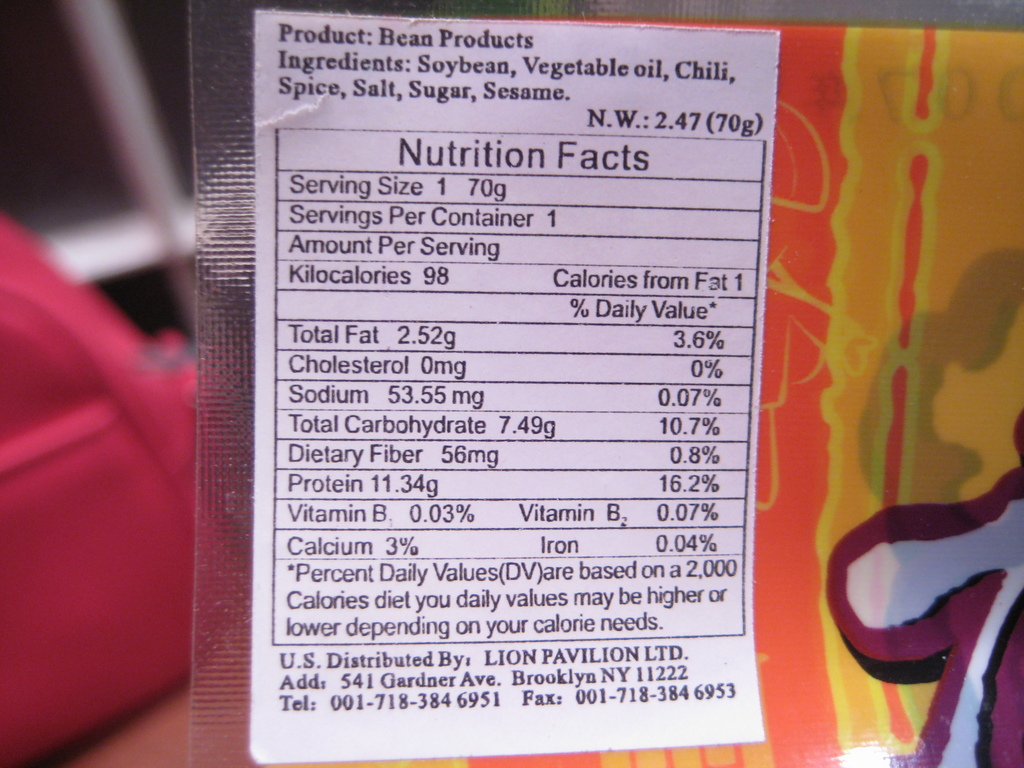This close-up image showcases a snack packaged in a striped orange and yellow plastic wrapping. The focus of the image is on the top left corner of the packaging, where a detailed Nutrition Facts label is prominently displayed. The label is enclosed in a white box and provides comprehensive nutritional information about the product, a type of bean snack. 

At the top of the Nutrition Facts label, the product is described as containing bean products. The ingredients listed include soybean, vegetable oil, chili, spice, salt, sugar, and sesame. The standard Nutrition Facts box indicates a serving size and servings per container, with a caloric content of 98 kilocalories per serving and 0% cholesterol. Notably, the protein content is 11.34 grams, accounting for 16.2% of the daily value. 

Additional information is found at the bottom of the label, including the distributor's details: Lion Pavilion, located at 541 Gardner Avenue, Brooklyn, New York, 11222. Contact information is also provided, featuring a telephone number and a fax number.